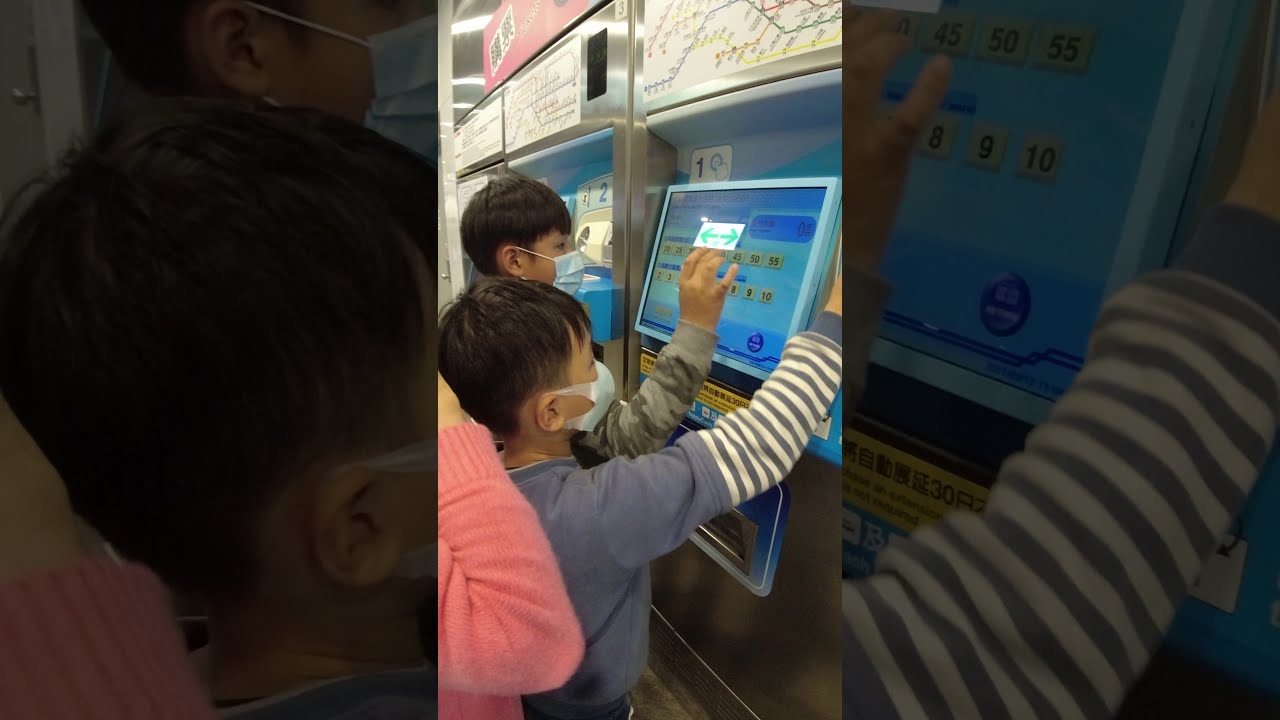This is a detailed photograph, possibly a screenshot from a video, of two children interacting with a touchscreen in what appears to be a subway station. The central focus is a vertically oriented image, where the surrounding borders are filled with zoomed-in and slightly blurred sections of the video, giving close-up views of the children's heads on the left and the screen on the right. The children, both wearing blue surgical face masks, are standing in front of a large monitor, which displays a range of numbers from 20 to 50 and includes green arrows for navigation. One child, dressed in green camouflage clothing, has a raised arm, actively touching the screen, while a second child, closer to the camera, wears a blue top with blue and white striped sleeves. Additionally, a third child’s arm, clad in a pink sweater, is visible on the left side of the image. The surrounding environment suggests this might be an indoor station area, possibly a spot where tickets are purchased, as indicated by what looks like a transit map on the blue screen and the children's engagement with it.